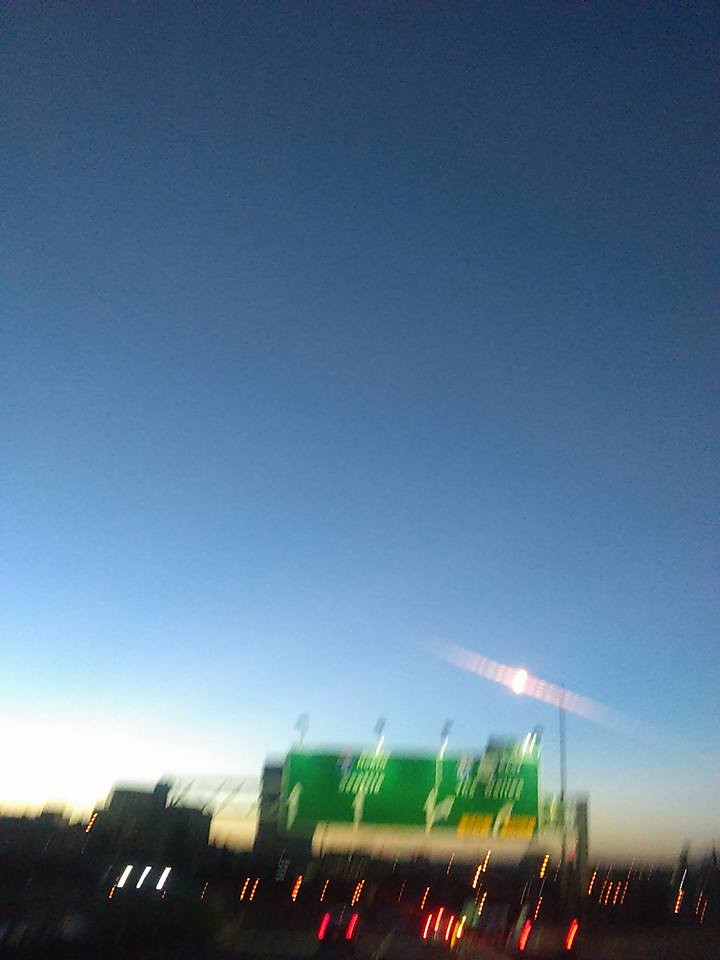A blurred photograph captures the dynamic scene of a journey on a highway during dusk. The upper portion of the image showcases a clear evening sky, transitioning from a darker shade of blue at the top to a lighter hue near the horizon, signifying the setting sun. The sky is cloudless and devoid of stars, emphasizing the twilight period. In the lower half of the image, numerous car lights illuminate the road, indicating heavy traffic. These lights create streaks due to the motion, accentuating the sense of speed and movement. A green highway sign is centrally positioned in the image, slightly below the midpoint; however, the text is unreadable due to the blur. The overall perspective suggests that the vehicle capturing the image is traveling northward.